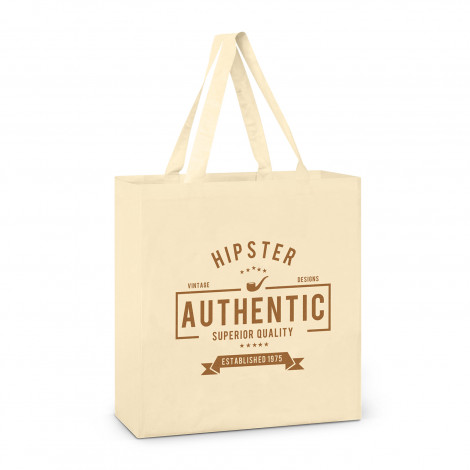This image features a light tan, rectangular cloth tote bag suspended against a plain white background, creating the appearance of it floating. The bag has two loose handles that extend upwards, suggesting it might be hung on an unseen hanger. The front of the bag prominently displays brown text and graphics. At the top, "Hipster Vintage Designs" is written in a semi-circle, with a pipe illustration just below "Hipster." Underneath, the words "Authentic Superior Quality" are centered within the design, flanked by five small stars. Below this, a banner with folded, V-cut ends reads "Established 1975." Overall, the detailed and vintage-inspired design hints at a product possibly showcased for online retail.